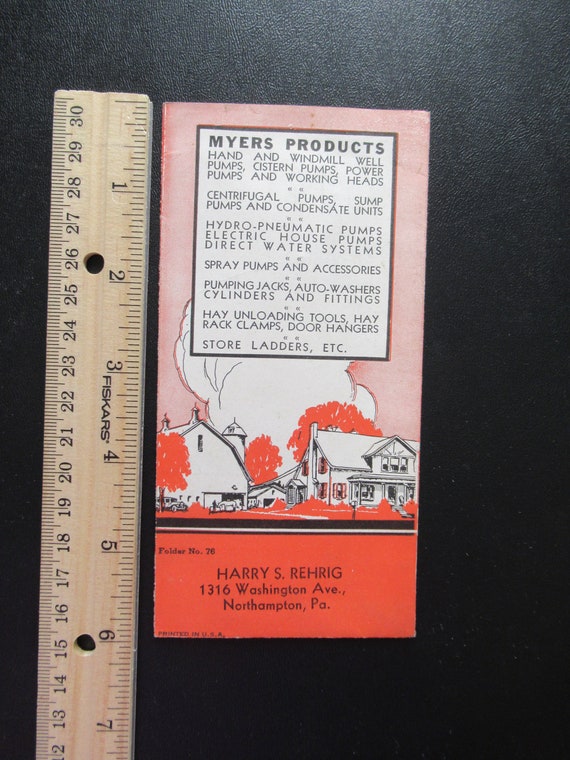The vertically rectangular, full-color image depicts a vintage advertisement booklet measuring 6 inches tall and approximately 4 inches wide, set against a dark wooden table or countertop. To the left of the booklet, a wooden ruler with markings from 1 to 7 inches helps to confirm its dimensions. The booklet, situated prominently in the center, features an illustration of a farm with a barn and a silo. The cover of the booklet states:

**"Harry S. Rehrig, 1316 Washington Avenue, Northampton, PA."**  
**"Meyers Products: Hand and Windmill Well Pumps, Cistern Pumps, Power Pumps"**

In fine print, the advertisement also lists various other products such as working heads, centrifugal pumps, sump pumps, hydro-pneumatic pumps, electric house pumps, hay unloading tools, hay rack clamps, door hangers, store ladders, spray pumps, and accessories.